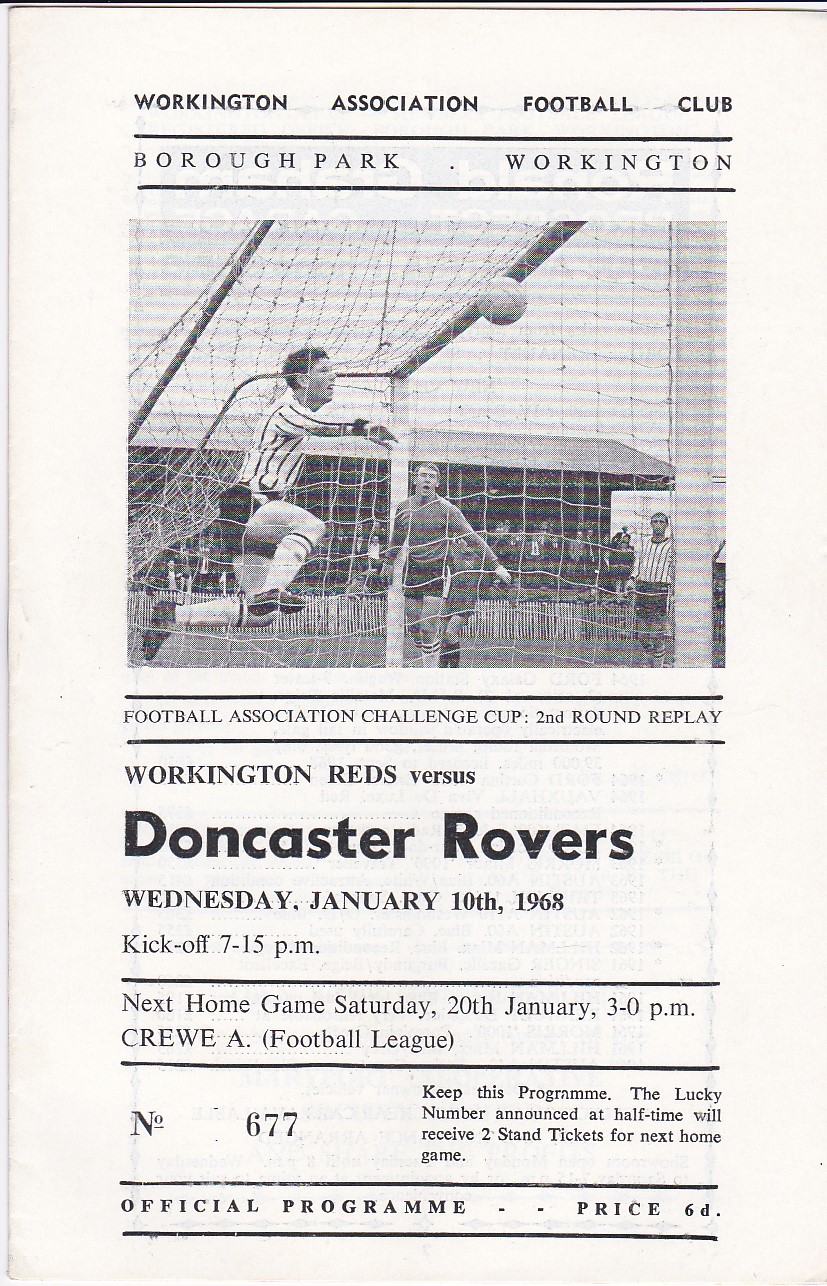This is a black and white page from an official football match program featuring an image of a goalie attempting to block a soccer ball from entering the net. The background shows other soccer players and a referee. Across the top, the text reads, "Workington Association Football Club, Borough Park, Workington." Below the image, the text details, "Football Association Challenge Cup, second round replay. Workington Reds versus Doncaster Rovers, Wednesday, January 10th, 1968." The kickoff time is noted as 7:15 PM. Additional information includes, "Next home game, Saturday, 20th January, 3 PM. Crew A Football League, number 677." The program instructs, "Keep this program. The lucky number announced at halftime will receive two stand tickets for the next home game." At the bottom of the page, it says, "Official Program, Price 6D." The entire page is filled with black text on a white background, separated by lines.